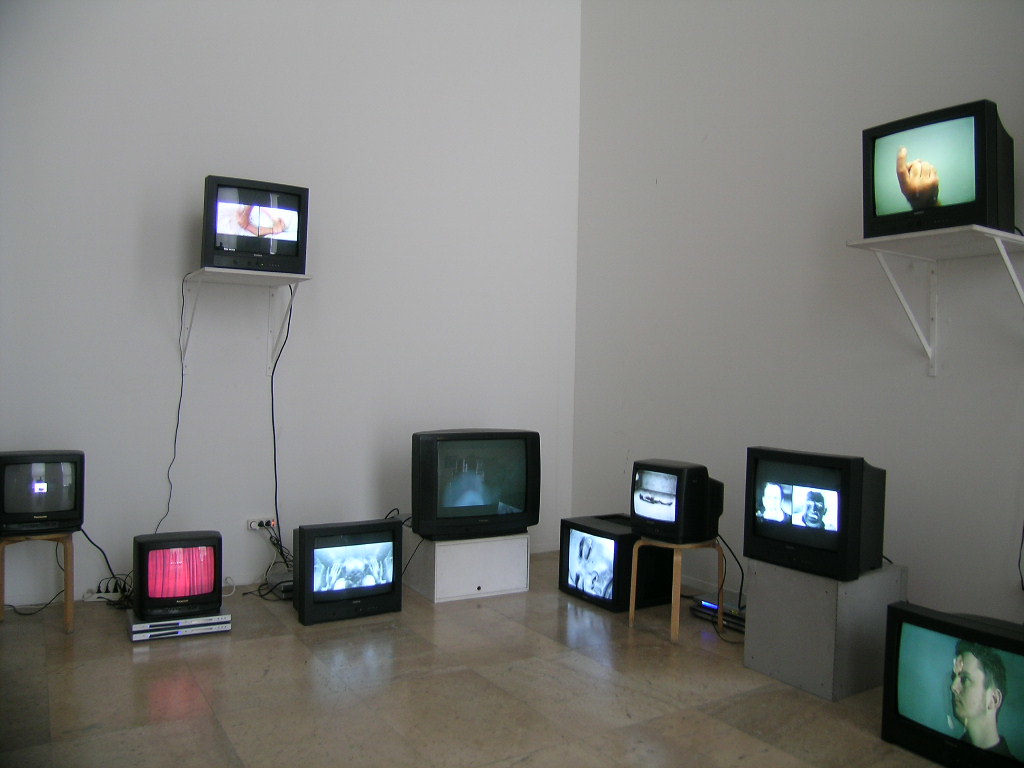The image depicts a room, possibly an art museum exhibit, with tall gray walls and a glossy tile floor in shades of tan and gray. Various old-style box TVs with glass screens are arranged throughout the space. On the left wall and side of the room, TVs are positioned on shelves, stools, and directly on the floor. One TV on the left is placed atop a DVD player, displaying bright curtains, while another on a stool shows an image of a person lying down. Further to the left, atop another shelf, is a TV with a pointing finger. 

On the right side, several TVs are placed on white cabinets and brown stands. The lowest TV to the right displays the side profile of a person, while another one on a stool shows x-ray imagery of people. High on the right wall, another TV features what appears to be a side-sleeping head. Multiple power cables and outlets are noticeable, connecting the TVs and contributing to a somewhat cluttered appearance with tangled cords. This array of differently positioned TVs projects various images, creating a diverse visual experience within the room.